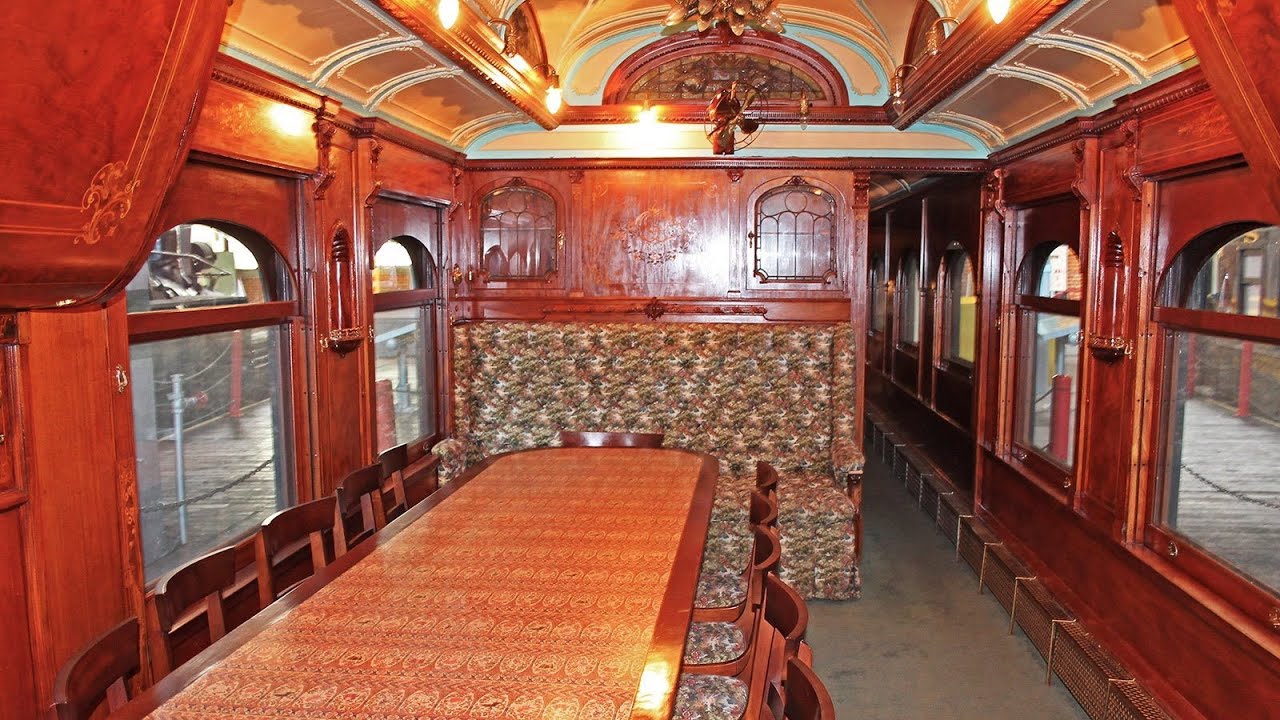This image captures the interior of an old-time train dining car, possibly from the 1800s. The elegant space is characterized by extensive use of beautifully polished hardwood, including a long oblong wooden table. The table is surrounded by numerous wooden chairs with floral-patterned cushions—seven on each side and one at each end, seating a total of 16 people. The ceiling, which is low and ornate, features a decorative woodworking dome and lights along the top. The interior is filled with a sense of warmth from the waxed and shiny wood surfaces. Large windows line the right side, extending down a hallway, while the left side has two windows near the head of the table. The detail and craftsmanship suggest a luxurious setting, enhanced further by views outside, which appear to include a dock with chains, hinting that this could also be part of a dining experience on a boat.